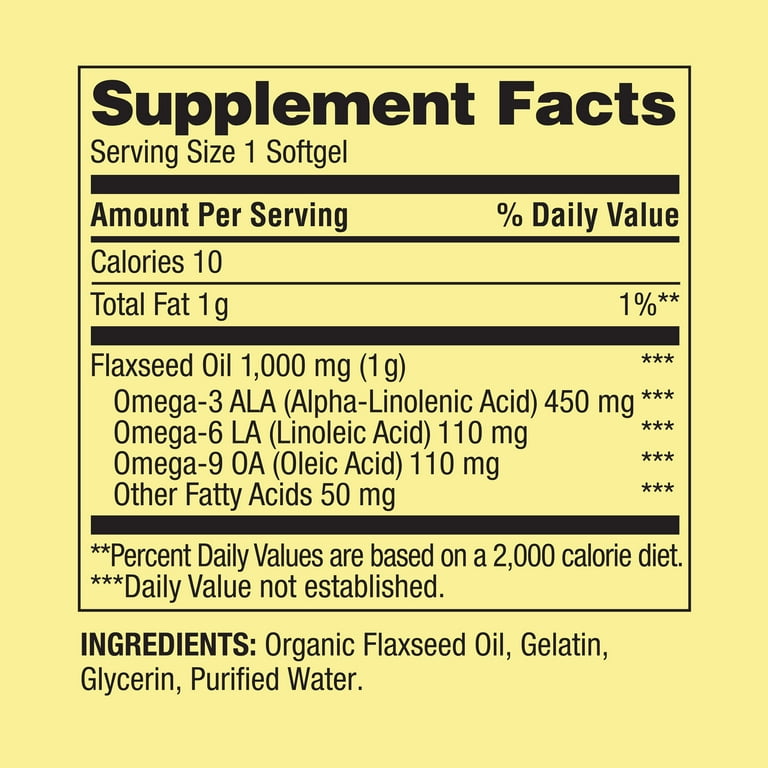This is an image of the ingredient panel and nutritional label for a bottle of flaxseed oil vitamin supplements. The label, in yellow and black, details the supplement facts and serving size, which is one soft gel. Each soft gel contains 10 calories and 1 gram of total fat. The primary ingredient is organic flaxseed oil, amounting to 1000mg per soft gel. This includes specific amounts of fatty acids: omega-3 ALA (450mg), omega-6 LA (110mg), omega-9 oleic acid (110mg), and other fatty acids (50mg). Additional ingredients listed are gelatin, glycerin, and purified water. The label is strictly the back panel and does not reveal the manufacturer's identity. The percent daily values are based on a 2000-calorie diet, although the daily value for these nutrients is not established. This supplement is intended for daily consumption for health benefits related to its omega fatty acid content.